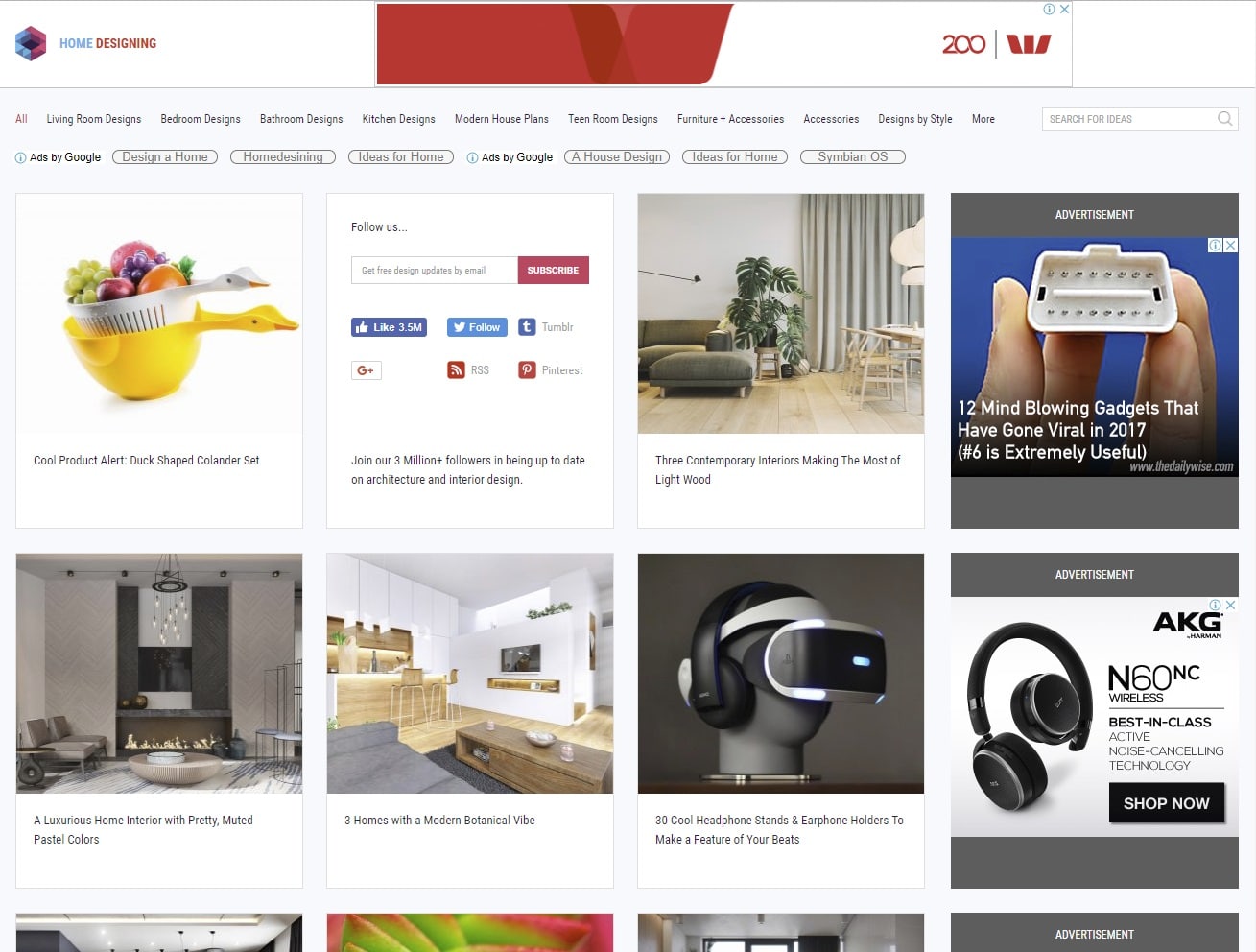**Top Left Corner:**

- Text: "Home Design"
  - "Home" in blue
  - "Design" in red
- On the right side of the text, there is a red bar
- Next to the red bar: "200 W"

**Bottom Area:**

- Tabs:
  - All
  - Living Room Designs
  - Bedroom Design
  - Bathroom Designs
  - Kitchen Design
  - Modern House Plans
  - Teen Room Design
  - Venture Plus Accessories
  - Accessories Designed by Style
  - More
  - Search box: "Search for ideas"

**Left Side:**

- Below Tabs: An ad from Google:
  - "Ads by Google"
  - Text: "Design a home, home designing ideas for home, house design ideas for home"
  - Another ad: "Simian OS"
- Below this:
  - Product: "Cool Product Alert: Dark Shaped Colander Set"
  - Description: The set is orange.

**Right Side of the Colander Set Ad:**

- Follow Us Section:
  - "Follow us: Get free design updates by email"
  - Red subscribe button: "Subscribe"
  - Social Media Icons: Facebook, Twitter, Tumblr, Google+, RSS, Pinterest
  - Text: "Join our 3 million+ followers in staying up-to-date on architecture and interior design"

**Middle/Right Side:**

- Image:
  - Description: "Three contemporary interiors making the most of light wood"
- Below that:
  - Text: "30 cool headphone stands and earphone holders to feature your beats"
- On the left side of that:
  - Image: "Three homes with a modern botanic vibe"
- Another left-side image:
  - Description: "A luxurious home interior with pretty muted pastel colors"

**Top Right Corner:**

- Advertisement:
  - "12 mind-blowing gadgets that have gone viral in 2017. Number 6 is extremely useful."
  - Website: dailywise.com

**Bottom Right Advertisement:**

- Product: "AKG N60 NC Wireless"
  - Description: "Best-in-class active noise-cancelling technology"
  - Button: "Shop now"
  - Image: Headphones by AKG